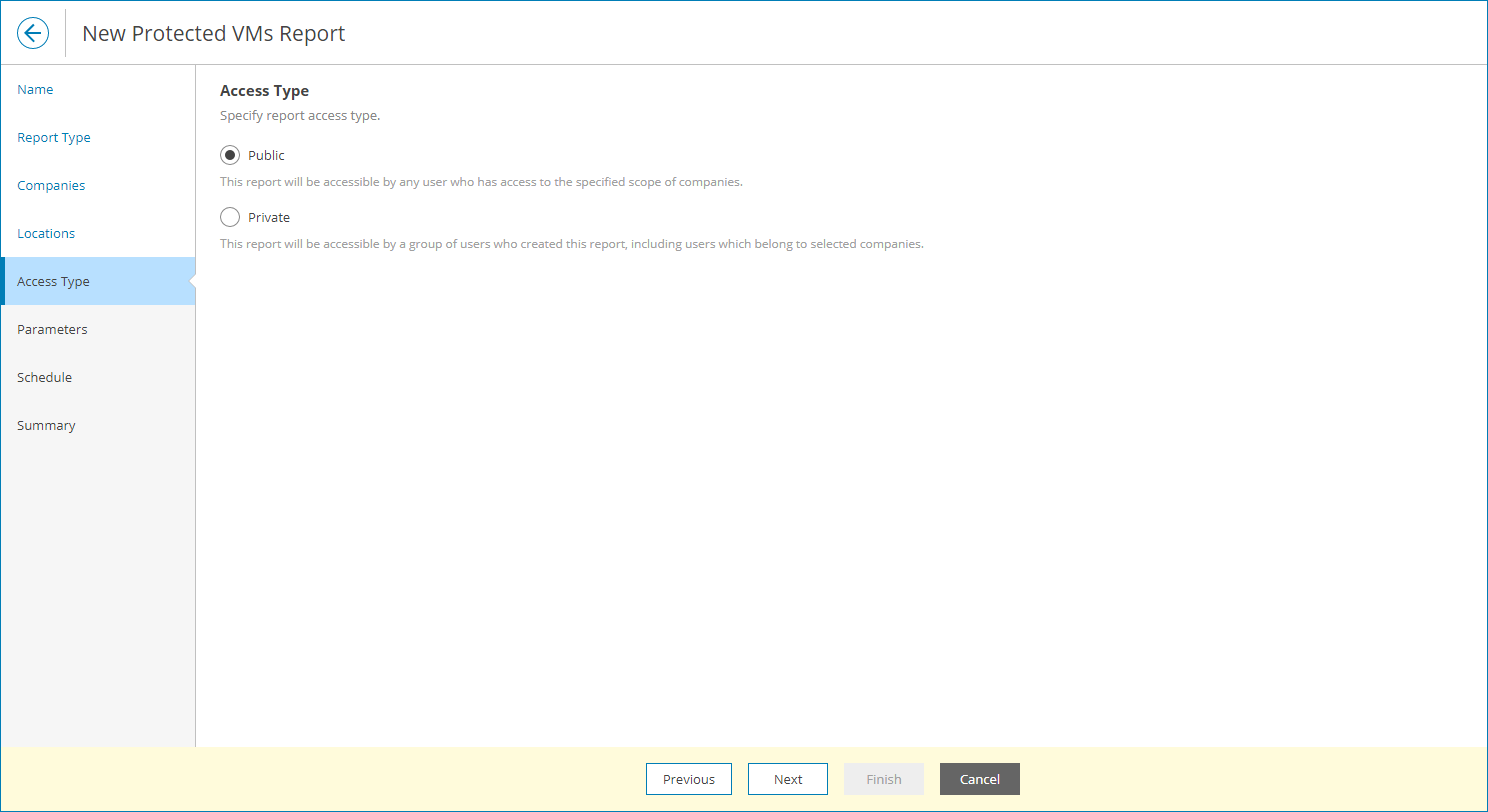The image is a rectangle with the longer side extending horizontally. It is bordered by a thin blue line that encloses the entire image. The main background is predominantly white, with a yellow border along the bottom. 

At the top of the image, there is a black arrow pointing to the left, followed by the text "New Protected VMS Report" in black letters. On the left side, a vertical column contains blue text that reads: "Name," "Report Type," "Companies," "Locations," "Access Type" (highlighted in blue), "Parameters," "Scheduled," and "Summary."

Adjacent to this column, in the main section of the image, black text details specific report access types:
- "Access Type"
- "Specify Report Access Type."
   - "Public: This report will be accessible by any user who has access to the specified usage of companies."
   - "Private: This report is accessible by a group of users who created the report, including users belonging to selected companies."

The yellow border at the bottom contains the navigation options presented in black text: "Previous," "Next," "Finish," and "Cancel."